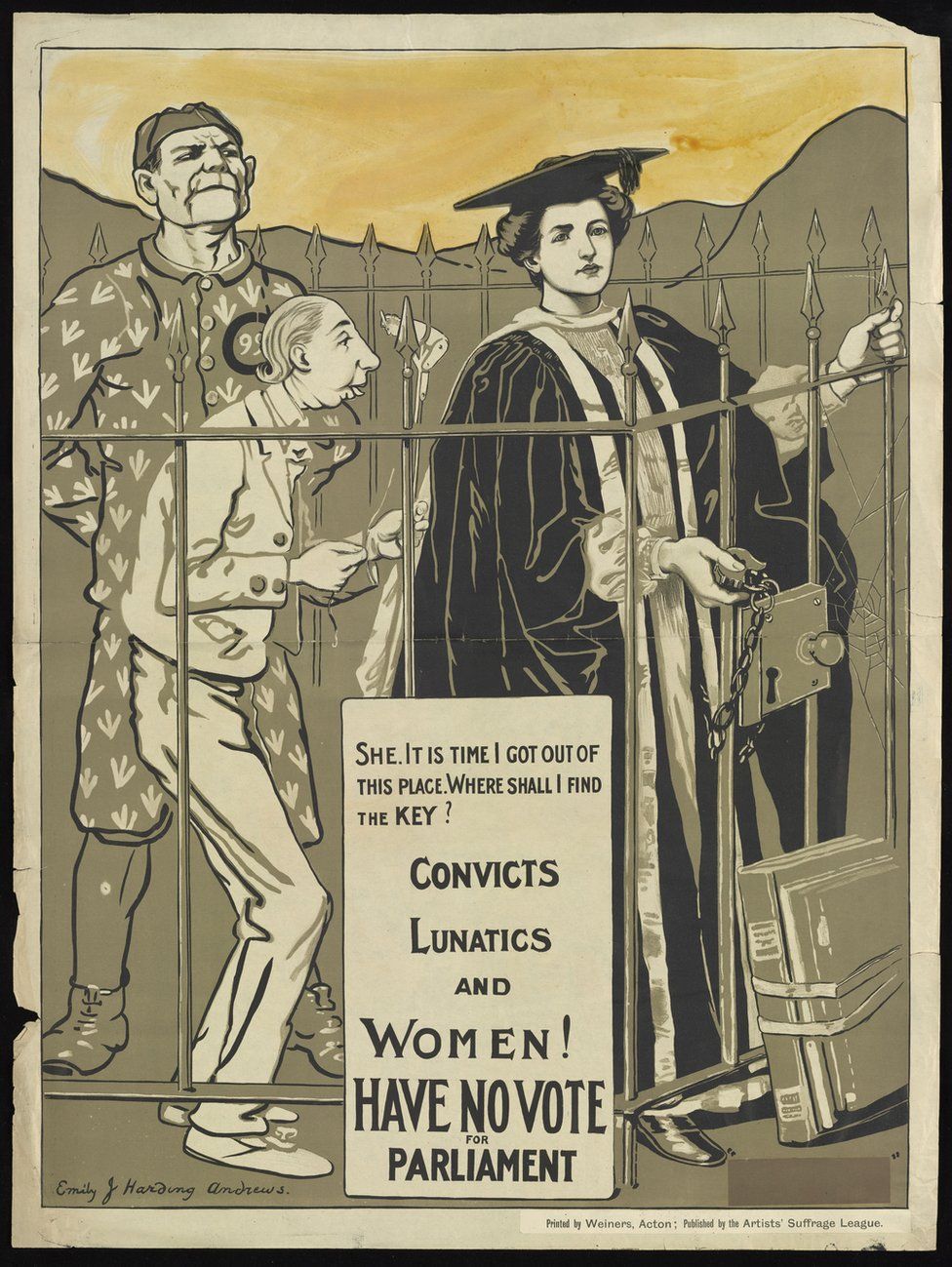This detailed poster, likely from the late 19th or early 20th century, serves as a political illustration promoting women's suffrage. It depicts three individuals behind a large wrought iron gate adorned with long spikes. The background features a watercolor sky painted in orange hues against large gray mountains. Prominently, there is a woman in the foreground with short curly hair, wearing a black graduation gown and cap, symbolizing a female graduate. Her hand extends through the bars, clutching a padlock outside the gate. Next to her on the right, a poster ominously declares, "She, it is time I got out of this place. Where shall I find the key? Convicts, lunatics, and women have no vote for Parliament."

Behind the woman, two men are visible. One man in the back right is dressed in a pajama top with a small cap, evoking the image of a convict. The other man stands next to him, clad entirely in white, adding to the somber tone. The edge of the poster features a black banner, framing the composition. This poignant and symbolic imagery underscores the message by the Artists Suffrage League, challenging the unjust denial of voting rights to women by likening their plight to that of convicts and lunatics.